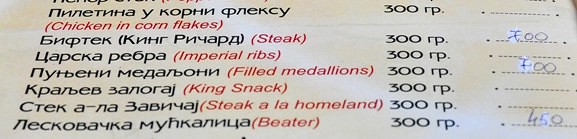This is a detailed photograph showcasing a section of a restaurant menu. The menu is divided into three primary columns. The left-most column lists various dishes in an unidentified native language written in black ink. Next to each dish, the English translation is provided in red ink and enclosed in brackets.

The first item listed is something akin to "Chicken in Cornflakes," which costs 300 RP. Following this, another dish is translated as "Steak," also priced at 300 RP. Other dishes in this column include "Imperial Ribs," "Filled Medallions," "King Snack," "Steak a la Homeland," and a dish called "Beater," each initially listed as 300 RP.

The second column indicates the price of each dish, initially marking them all at 300 RP. However, there are notable corrections made using white-out (TPEX). For example, the prices for "Steak" and "Filled Medallions" have been updated to 700 RP, with the original numerals covered with TPEX and rewritten. Similarly, the price for "Beater" has been altered to 450 RP, with the '5' written over the white-out.

The third column consists of dotted lines, presumably for additional notes or adjustments. There are handwritten prices alongside some specific dishes: "Steak," "Filled Medallions," and "Beater," indicating the updated prices of 700 RP and 450 RP respectively. It seems these corrections reflect recent price adjustments on the menu.